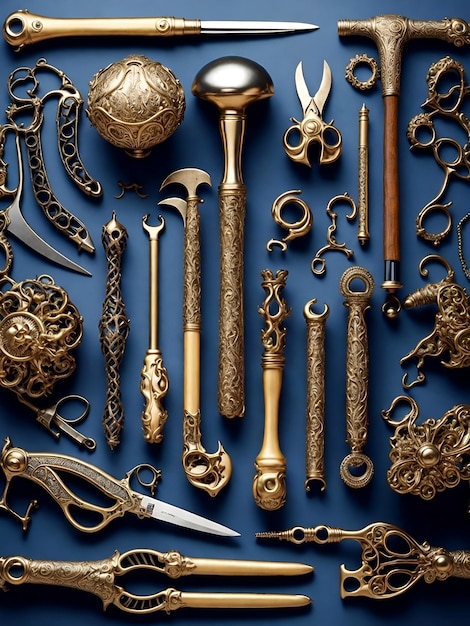This vertical rectangular image showcases a collection of tools and decorative items, evoking an olden, possibly medieval era. The background is a dark blue, and the items appear meticulously arranged. At the top of the image, there's a brass letter opener followed by a hammer with a brass top and a wooden handle. The tools, predominantly brass with varying degrees of shine, include hammers, picks, scissors, and pliers. Some items have intricately decorated handles, while others are more utilitarian. Additionally, there are objects resembling hinges or decorative elements, possibly for a wooden chest. The background, which resembles a soft material like velvet but appears somewhat grainy, may be intended to contrast with the metallic sheen of the tools. This array of implements, some appearing as potential weapons such as stilettos and ornamented knives, combine practicality with decorative artistry.